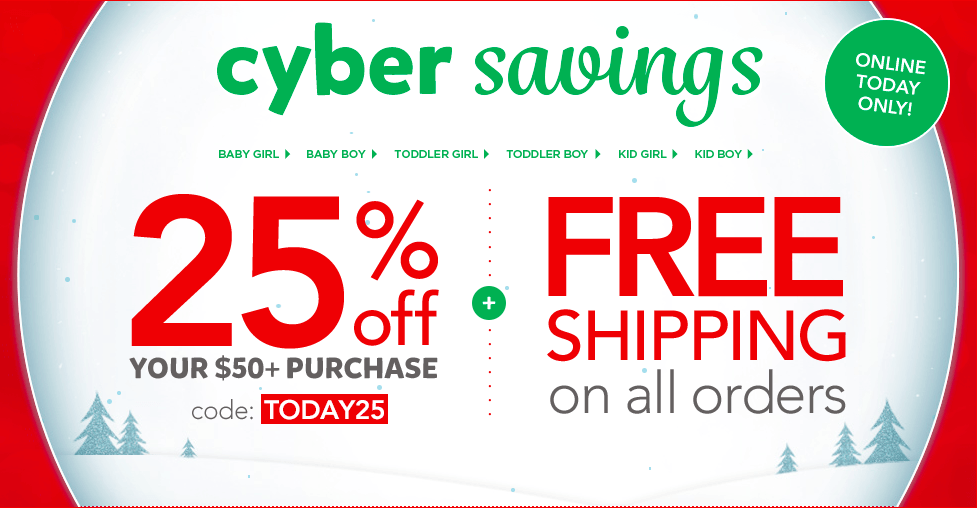Screenshot of a festive promotional graphic titled "Cyber Savings." The design features a large white circle resembling a snow globe, flanked by red borders. Inside the circle, "Cyber Savings" is written in green text. The deal highlights include 25% off for various categories such as baby girl, baby boy, toddler girl, toddler boy, kid girl, and kid boy. A red dotted line runs across the graphic with a green solid circle featuring a plus sign in the middle. There's an offer for free shipping on all orders, and a special $50+ purchase code "TODAY25" written in a red box. The background is adorned with images of snow and green pine trees reminiscent of Christmas, and the entire graphic is enclosed within a red dotted border.